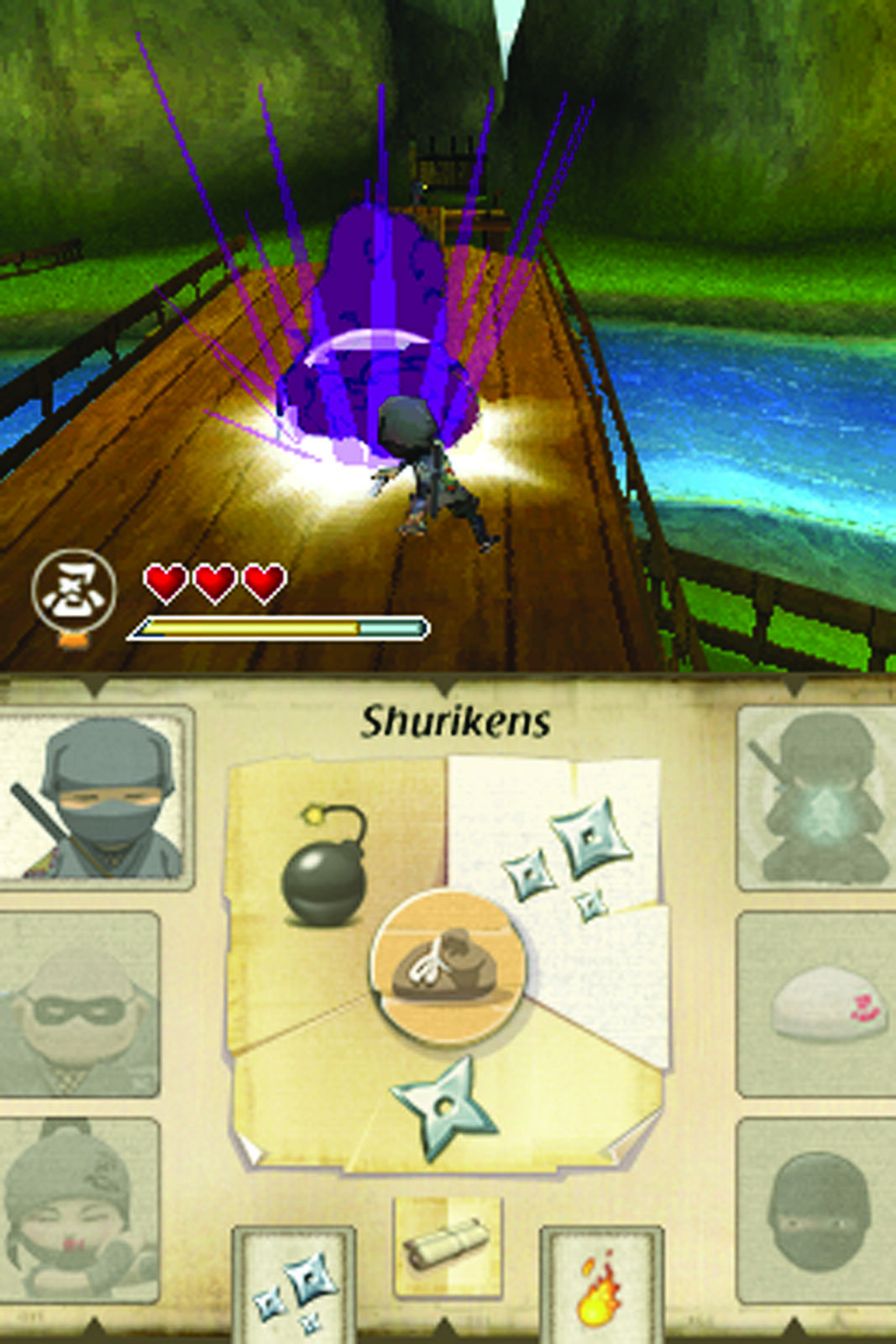This vivid and cartoonish screenshot from a fighting video game showcases a dynamic scene centered on a brown, dark-rimmed bridge spanning a river with vibrant fluctuating shades of blue. The protagonist, a ninja-like character clad in dark and light grey, battles a monstrous purple glob accented with pink and violet streaks. As the ninja strikes, star-like bursts of light materialize around the creature. The bridge scene is flanked by lush green grass and towering dark and light green mountains, giving an impression of a serene environment juxtaposed with the ongoing combat.

Above the bridge, vibrant green foliage and bright emerald lawns hint at a forest setting. The top of the image is adorned with a heart bar interface, displaying a white-bordered bar transitioning from yellow to blue, with a silhouette encircled by red hearts, indicative of the ninja's life status.

The bottom section of the screen is dense with interactive elements. There are six selectable icons representing the ninja’s arsenal, including shurikens, a bomb with a lit fuse, throwing stars, a map, a fire button, and various character icons. Each icon is meticulously detailed with highlights and shadows, creating a visually rich user interface. In particular, the shuriken icon, spelled out in black text as "Shurikens," stands out prominently at the top. Other icons include a paper scroll, a tan and orange square, and a satchel with a white string, each contributing to the immersive experience with their distinct designs.